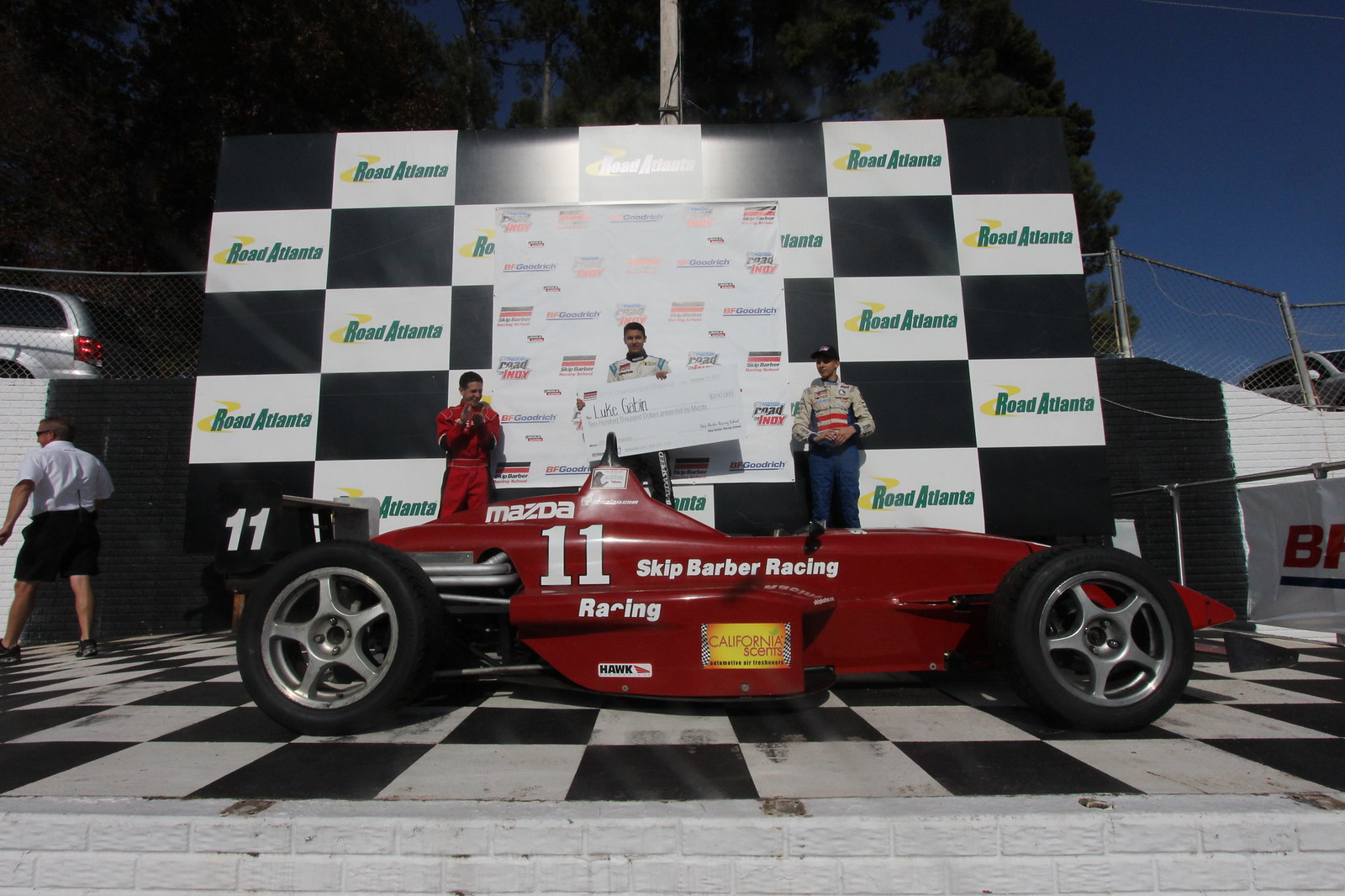The photograph captures a jubilant moment at a press event following a race, presumably held at Road Atlanta. The focal point is a distinctive red race car, sporting the number 11 and marked with "Skip Barber Racing" in white letters. This squat, open-cabin car, which also displays "Mazda," rests on a black-and-white checkered flag pattern, symbolizing its victory. Standing proudly behind the car is the apparent winner, Luke Gabbin, dressed in a white racing uniform and holding up an oversized check for $200,000. He is beaming with joy. To his right, a man in a red jumpsuit claps in celebration, while another individual in a racing suit stands to his left, potentially members of his pit crew or fellow racers. The backdrop features a press banner adorned with multiple logos, including "Road Atlanta," and has a similar checkered design. The event unfolds under clear daylight, adding to the clarity and vibrancy of this triumphant scene.